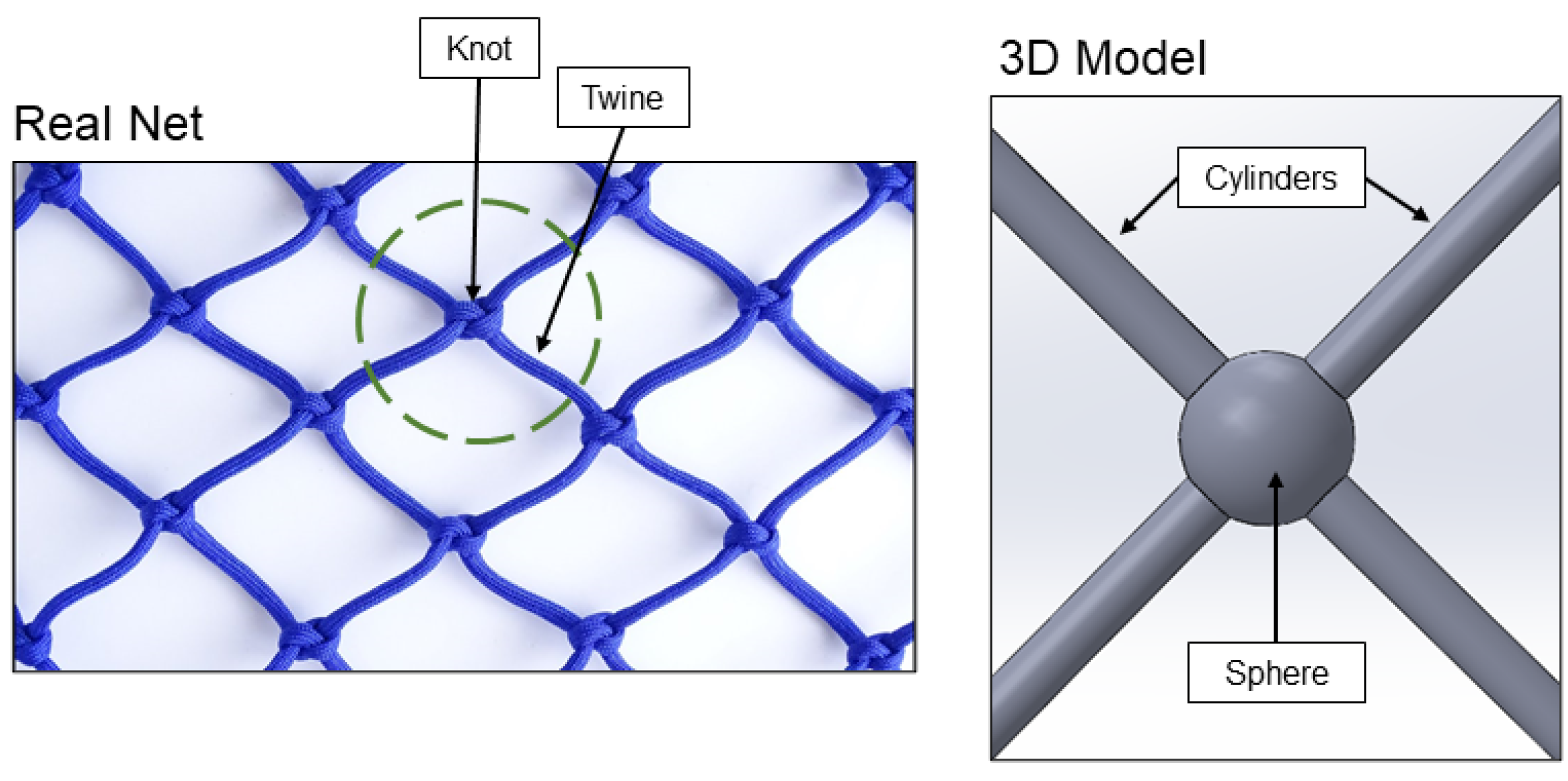The image comprises two side-by-side panels, each with a detailed focus on a netting structure. The left panel, bordered in black with a white background, is titled "Real Net." It showcases a blue net that resembles chain-link fencing. A dashed green circle highlights a central knot within the netting, with two labeled arrows pointing to key components: the "knot" and the "twine." The right panel, also outlined in black, is labeled "3D Model." This section features a 3D graphic composed of a central sphere with four gray cylinders extending from it in an X-like arrangement, illustrating the netting structure's connections and mimicking the real net shown on the left.